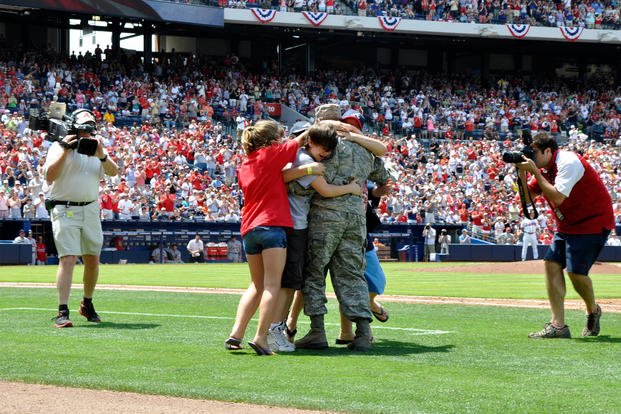The photograph captures a poignant scene at a baseball game, focusing on an emotional family reunion. The central figure, dressed in a military camouflage uniform, is warmly embraced by a young boy clinging to him and a woman in a red top with jean shorts, possibly his wife. Another family member, whose face is obscured, joins the hug from the side. The background shows a stadium filled with standing, applauding fans whose faces are blurred, indicating their shared joy and support. Americana bunting adorns the upper-level railing, adding a patriotic touch to the setting. On the right, a person with a camera in a red t-shirt and jeans photographs the touching moment, while another individual in a white outfit records the event with a video camera from the left. A baseball player and the expansive field add context to the setting, making it clear this heartfelt reunion took place during a special moment at the game.